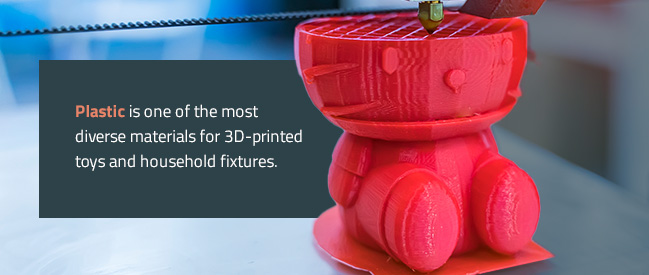This advertisement showcases the versatility of plastic as a material for 3D printing, specifically for toys and household fixtures. The image prominently features a 3D-printed red plastic figure resembling a sitting character, reminiscent of Hello Kitty with its squat legs, short arms, and distinctive facial features like whiskers and a button nose. Notably, the character's head is bowl-shaped, deviating from a human-like form, and appears to have a green screw attached to a metal rod over it. The character sits against a background speckled with white flecks, possibly depicting a room or office environment. Accompanying the image is a text blurb in mostly white font, with the word "plastic" highlighted in a light shade of orange. The text reads: "Plastic is one of the most diverse materials for 3D printed toys and household fixtures." This statement is placed within a grayish rectangular block that extends from the side of the character's body.